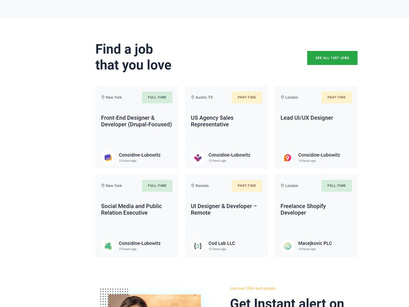This is a cropped screenshot of a job search website’s interface. The header on the top left reads, "Find a job that you love." Adjacent to this, on the right, is a prominent green button labeled "See All Jobs." Beneath the header, the webpage features six job listings arranged in two rows of three. Each job listing is enclosed in a gray square.

In the top left corner of each job listing, the location is displayed. The employment type of each job is indicated on the top right corner with colored bars—blue for full-time positions and yellow for part-time ones. There are three listings for each employment type. The central part of each box prominently features the job title, and the bottom of each box lists the respective company.

The background of the webpage is predominantly white, giving a clean and uncluttered look. At the very bottom of the cropped image, there is a partial view of some additional elements: a small image positioned to the left and a text snippet to the right that reads, "Get instant alert on," however, both the image and the text are partially cropped and not fully visible.